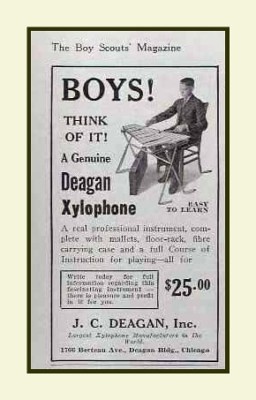This black-and-white vintage advertisement, likely from the Boy Scouts magazine, showcases an offer for a genuine Deegan xylophone. The advertisement is set against a cream or eggshell-colored background and features a boy seated in a chair playing the xylophone. The detailed picture displays the xylophone with its accessories, including mallets, a floor rack, and a fiber carrying case, neatly placed beneath the instrument. The header reads "The Boy Scouts Magazine" with an enticing call to action: "Boys, think of it! A genuine Deegan xylophone, a real professional instrument, complete with mallets, floor rack, fiber carrying case, and a full course of instruction for playing, all for $25." Additionally, the advertisement highlights "JC Deegan Inc., Largest xylophone manufacturer in the world," although the address, noted to be in Chicago, is too small to read. The boy in the image appears to be wearing a suit, adding to the professional allure of the instrument.